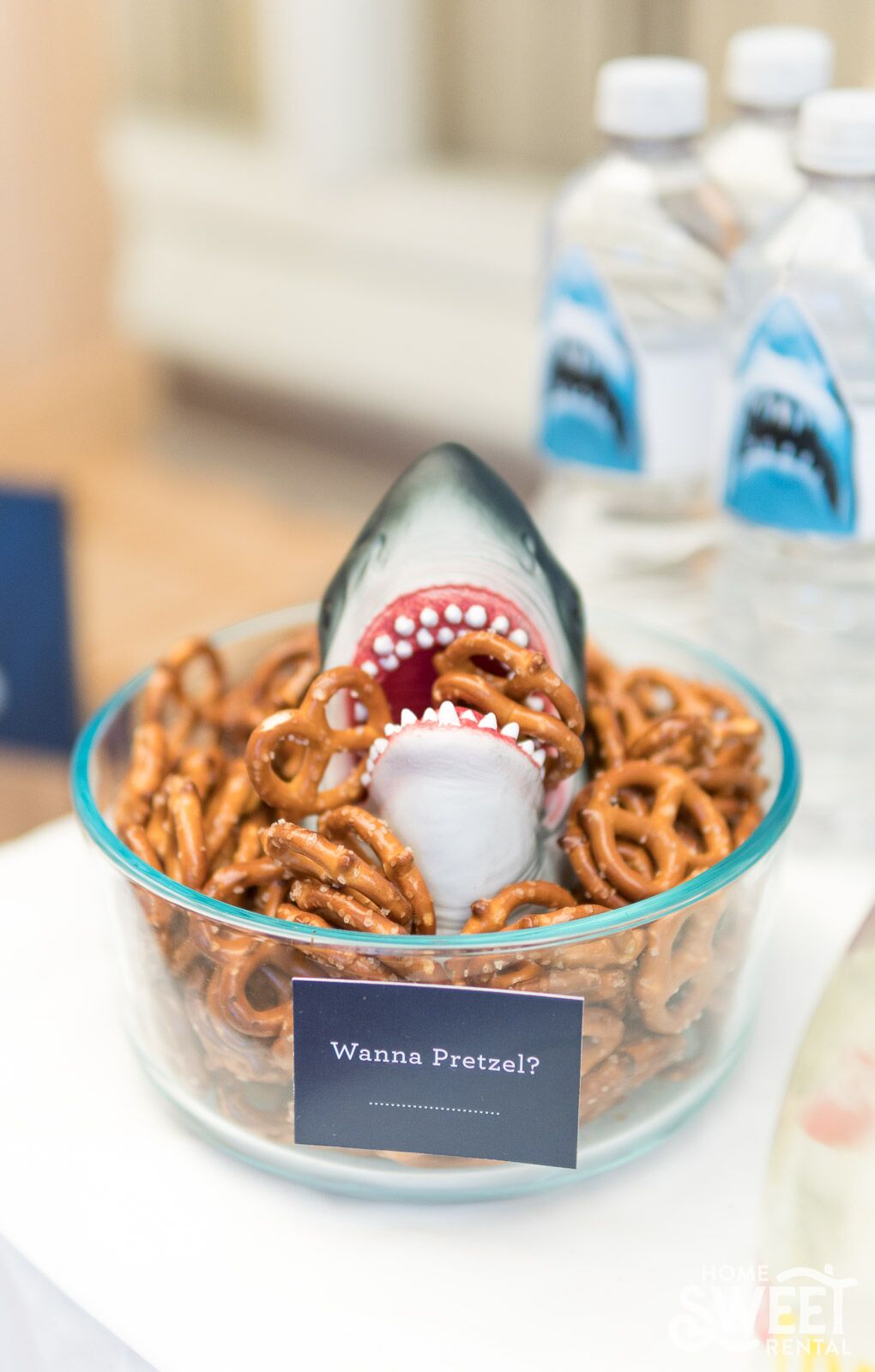In this whimsical photo, a clear glass bowl, possibly made of Tupperware, is filled with pretzels. Dominating the bowl is a toy shark head, artistically placed to appear as if it is munching on the pretzels, with several bits of the snack in its mouth. Affixed to the front of the bowl is a black card with white, capitalized lettering asking, "Want a Pretzel?" beneath a thin horizontal white line. Surrounding this setup, on a hardwood floor with a white wall in the background, are clear water bottles featuring blue shark illustrations and white caps. The humorous and creative arrangement seems to playfully mimic a shark attack on the pretzels, possibly as a nod to Shark Week or a similar theme.